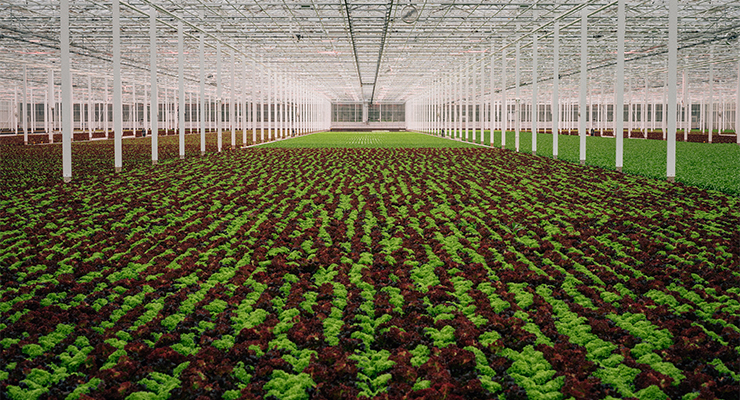The image depicts a massive commercial greenhouse or indoor plant production area, sprawling over an estimated two or three acres. The structure is bathed in natural light streaming through a glass ceiling supported by white columns and intricate metal scaffolding. The spacious, high-ceiling interior, at least two stories tall, features rows upon rows of small leafy plants—likely lettuce—with alternating bands of green and red foliage. The floor is a patchwork of green vegetation interspersed with brown dirt or gravel. In the foreground, green plants with red-brown tips dominate, extending into the background where even more neatly organized rows of vegetation continue as far as the eye can see. The bright white and green color palette is occasionally interrupted by the stainless steel of overhead pipes and ceiling fans. There is a slight variation in plant density, with thicker, fully-grown plants appearing on one side and less mature vegetation on the other. The orderly arrangement and the extensive infrastructure allude to a sophisticated, large-scale agricultural operation focused on optimizing plant growth indoors.